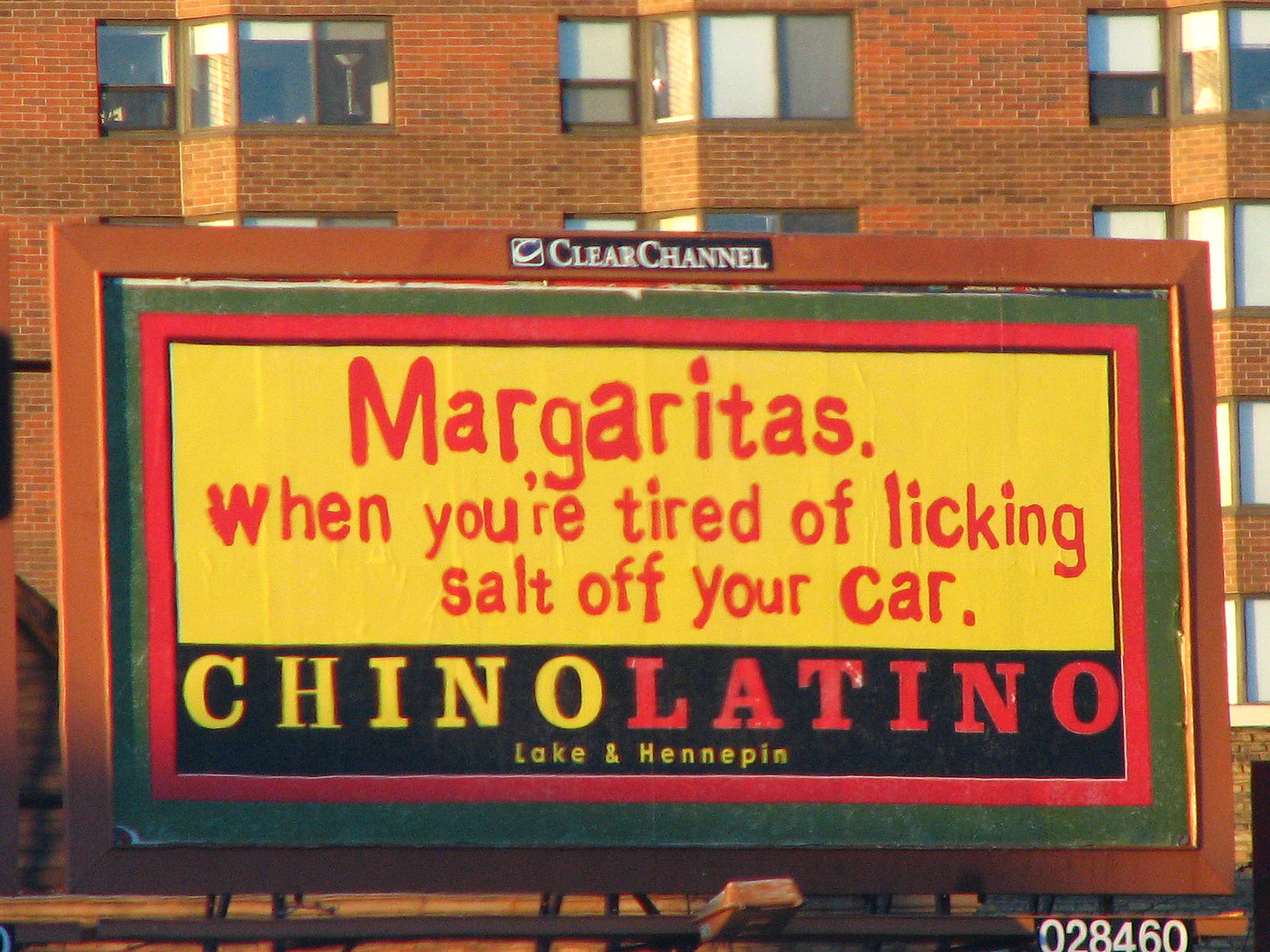This daytime outdoor photograph prominently features a large billboard with a rustic aesthetic and a complex visual configuration. The billboard displays a humorous message in a handwritten-style red font against a vibrant yellow background, reading, "Margaritas. When you're tired of licking. Salt off your car." Below this, a black horizontal strip contains the text "Chino Latino" - with "Chino" in yellow and "Latino" in red - and the location "Lake and Hennepin" in smaller yellow text. Additionally, a series of numbers, "028460," can be seen towards the bottom. The billboard is framed by brown, dark green, and dark red borders. It is branded with a "Clear Channel" logo in white on a black background at the top. An old, rusted light fixture, intended to illuminate the billboard at night, is visible at its base. In the background, a tall, slightly undulating brick building with multiple windows, indicative of residential or commercial use, adds a contextual backdrop to the scene.